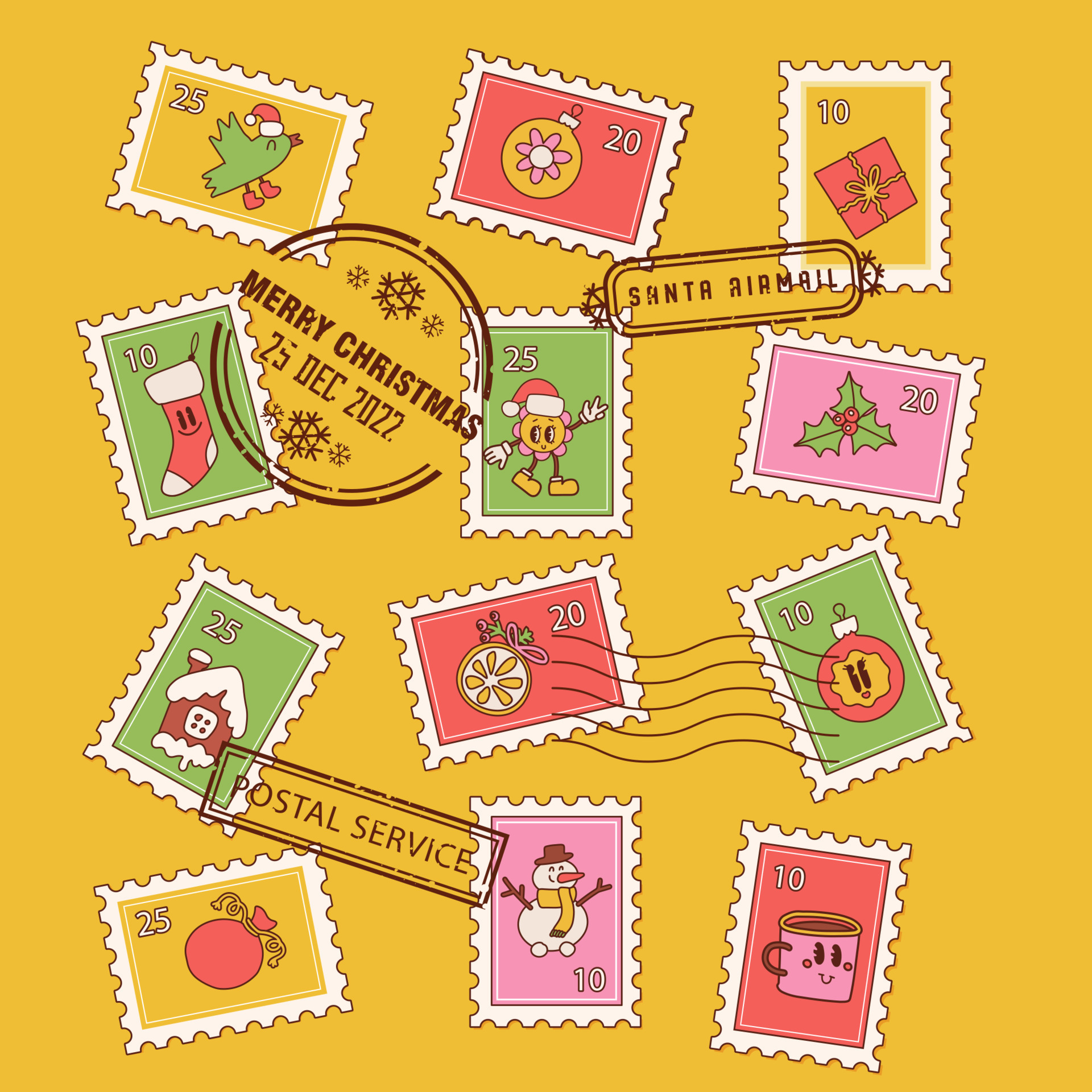The image displays a collection of 12 digitally illustrated, cartoon-like postage stamps set against a yellow background, each bearing Christmas motifs and numerical values. At the top left, there's a green bird adorned with a red Santa hat and boots, sitting in a yellow rectangle with the number 25 in white. To its right, a red rectangle holds a yellow ornament decorated with a pink flower and the number 20, while the top right features a yellow vertical rectangle displaying a red gift box with a yellow ribbon and the number 10. The second row begins with a green stamp showing a red stocking and the number 10, followed by a comical stick-figure Santa Claus on a red background labeled 25, and a piece of holly on a pink backdrop with the number 20. The third row includes a red house covered in snow on a green background marked 25, a round yellow ornament on a red field with the number 20, and another ornament, round and green, against a green background stating 10. The bottom row starts with a yellow background featuring a tied red bag and the number 25, followed by a snowman on a pink background with the number 10, and concluding with a pink mug with a smiley face on a red background. Overlapping the stamps is a post office cancellation mark reading "Merry Christmas 25 December 2022," enhanced with additional stamps labeled "Santa Airmail" and "Postal Service." The overall theme is festive, celebrating Christmas with whimsical, charming designs.